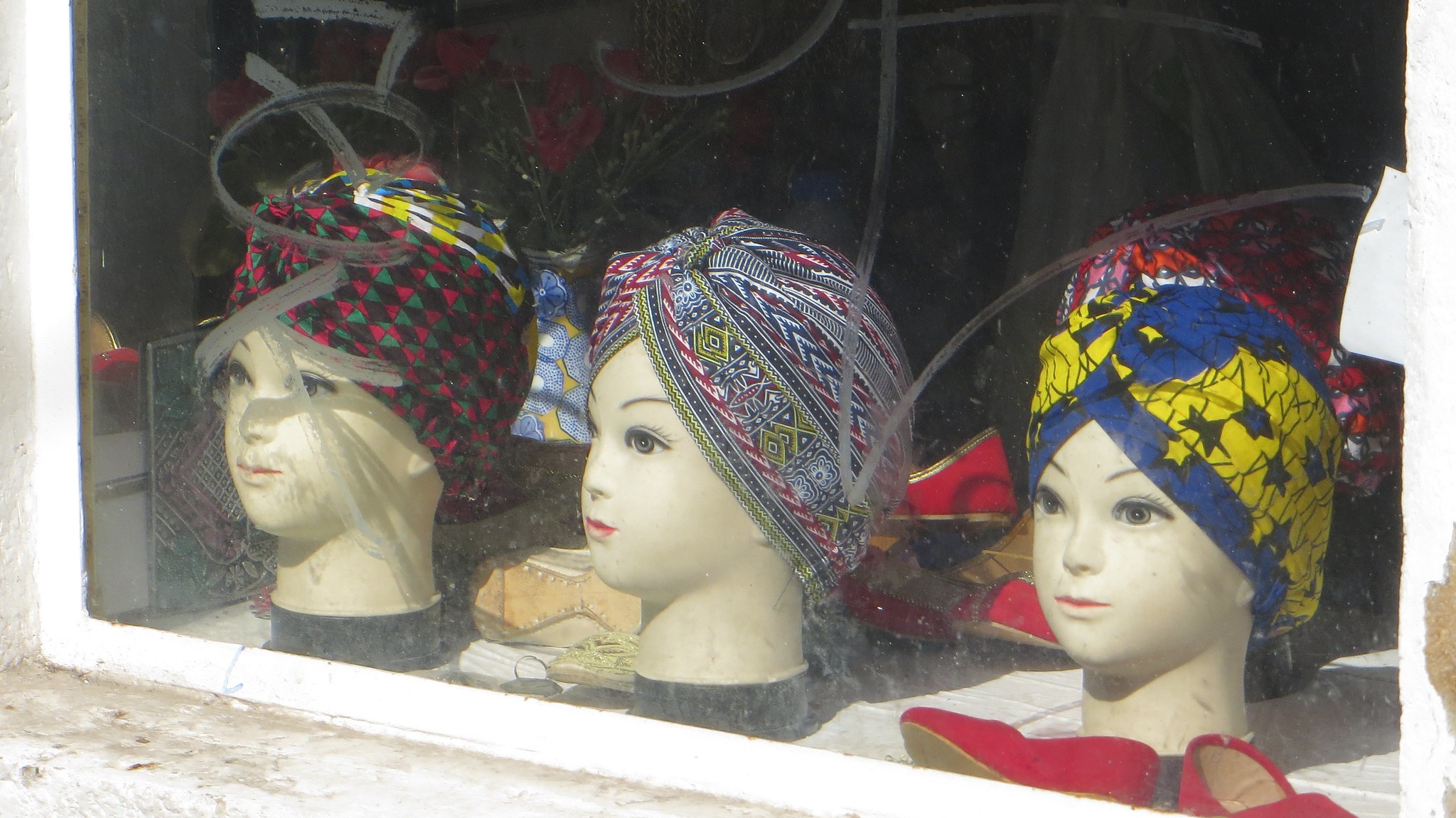A detailed close-up photograph of a shop window showcases three mannequin heads, each adorned with elaborate head scarves. The window, edged with a plain white border, displays Chinese writing on the left side, with a prominent large Chinese character on the right side. Through the window, a blue vase with red roses is slightly visible to the left, set against a dark interior. In front of the mannequins, there's a pair of red ladies' shoes—one positioned upright and the other on its side.

The three heads, arranged from left to right, appear identical with pale skin, bright red lips, and thin eyebrows, gazing leftward. The leftmost mannequin is adorned with a striking scarf featuring an intricate diamond pattern in red, green, and brown hues. The central mannequin sports a scarf with a multicolored, striped design, showcasing vivid sections of blue, yellow, and turquoise stripes interspersed with stars and more complex patterns of red, white, and blue. The rightmost mannequin’s scarf displays a simpler yet bold pattern of alternating dark blue and bright yellow stars, with an additional scarf showing hints of pink, orange, and white mixed in. The scene is accented by visible shadows and obscured objects in the background, adding to the depth and intrigue of the image.